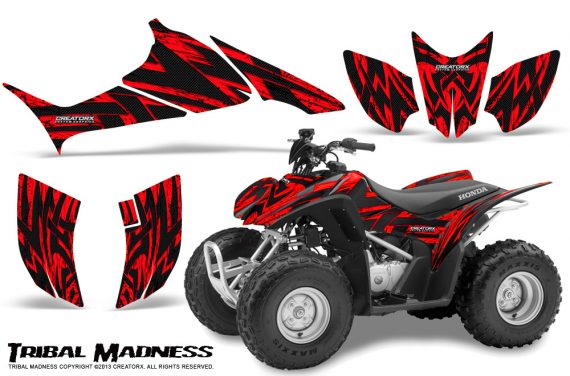The promotional image for the ATV highlights a red Honda quad bike prominently positioned in the bottom right corner. The ATV features intricate black tribal tattoo-style patterns over its red body, complemented by large black tires with silver rims. The seat, marked with the white text "Honda," sits above a visible silver and black engine. The front of the ATV showcases a rounded silver frame. Surrounding the main image of the ATV, the top and left sides display detailed close-ups of various body panels showcasing their textures and designs. Text in the bottom left corner reads "Tribal Madness" and includes a copyright notice: "Tribal Madness Copyright 2013 Creator X. All rights reserved." The overall arrangement and vivid colors present a balanced and engaging advertisement for the all-terrain vehicle.